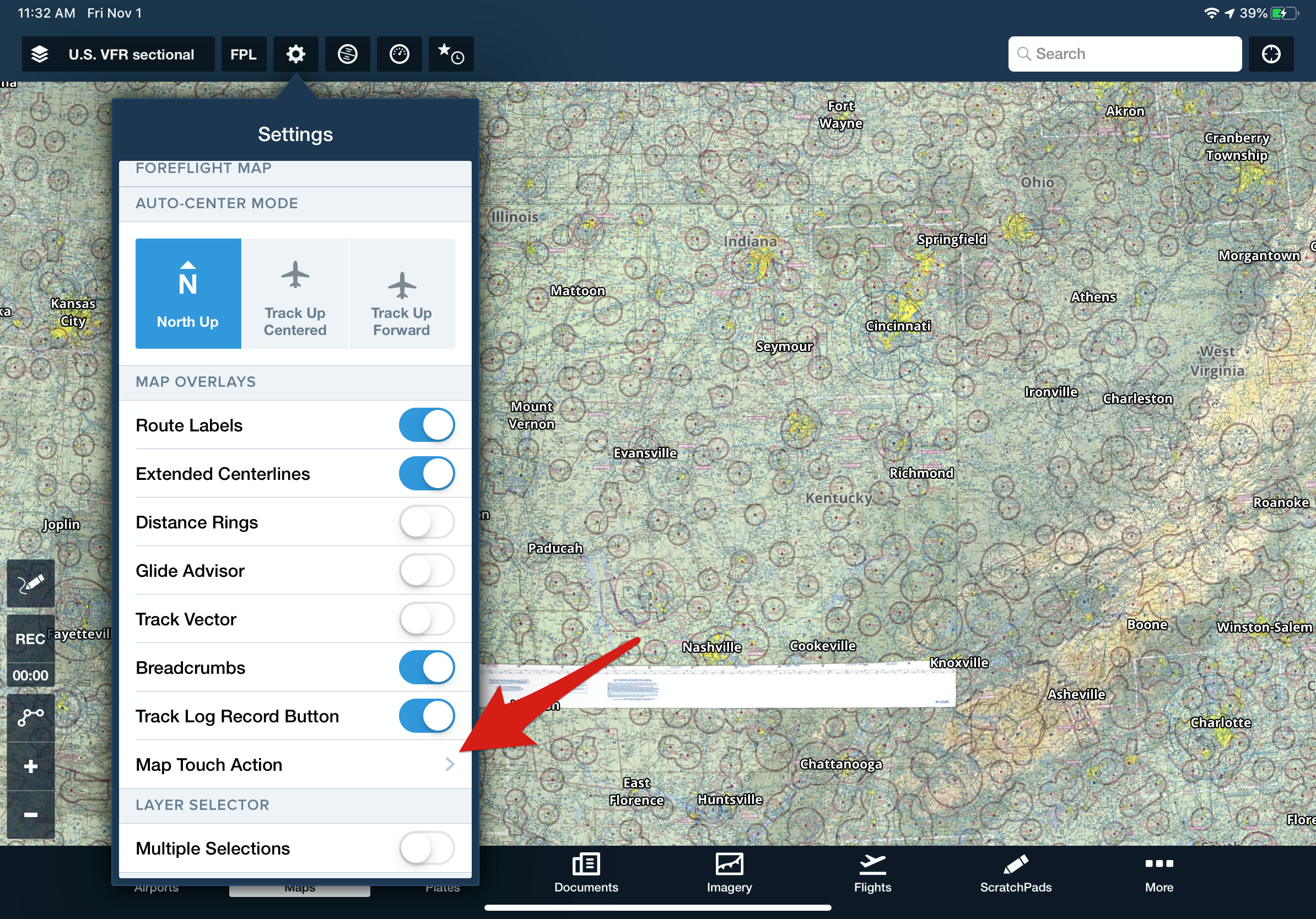The image is a screenshot of the settings section on a website or GPS application. At the top left corner, there's a pop-up window labeled "Settings." Below that, various configurable options are displayed. The first visible setting is "ForeFlight Map," followed by "Auto Center Mode," which offers several options including "North Up," "Track Up Centered," and "Track Up Forward." Following these, under "Map Overlays," the options "Route Labels" and "Extended Center Lines" are both enabled.

Further down, the settings "Distance Rings," "Glide Advisor," and "Track Vector" are turned off, whereas "Breadcrumbs," "Track Log," and "Record Button" are activated. Notably, there's a red arrow pointing toward the "Map Touch Action" option, indicating its significance or suggesting it as a focal point for the viewer. This detailed layout helps in understanding the various mapping and tracking functionalities available within the application.